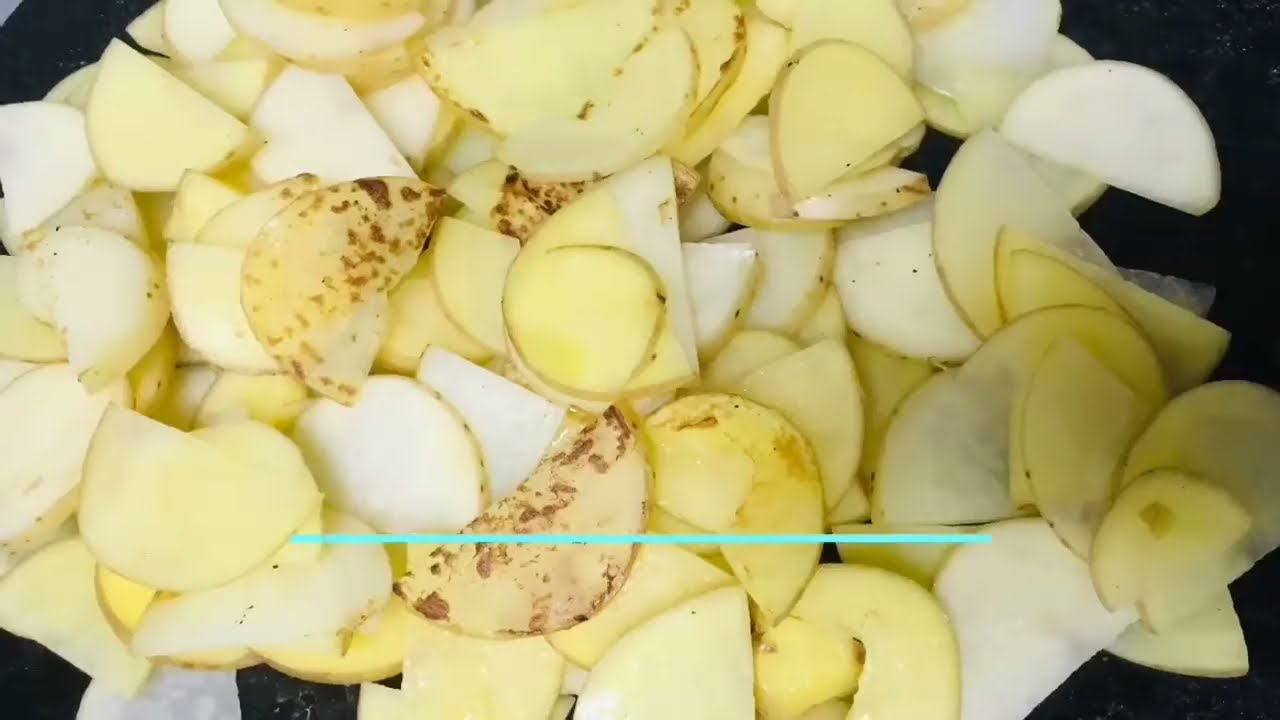The image depicts a substantial pile of varied potato slices, predominantly cut into half-circle shapes. The slices exhibit a range of colors from white to yellow, some featuring brown spots or patches, primarily on the skins. These potato slices are arranged on a circular black plate or surface, creating a scattered and overlapping display. Across the bottom of the image, nearly occupying half of the frame, there's a thin, horizontal aqua green line cutting through the center.